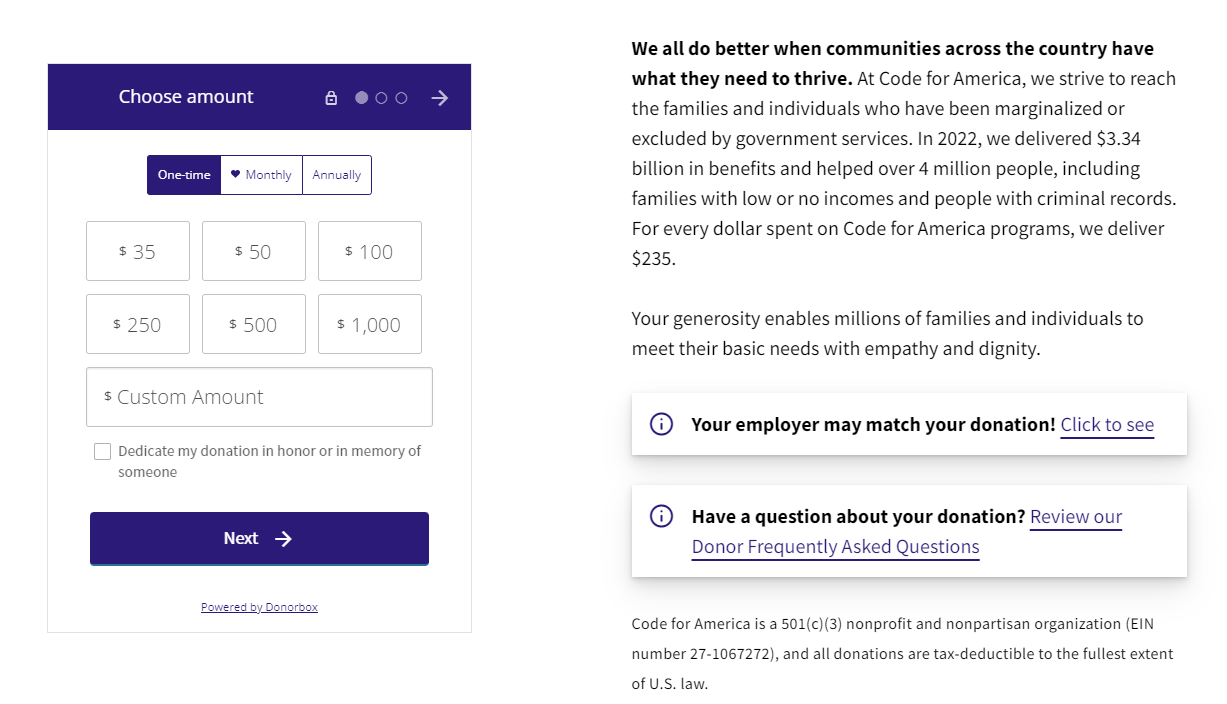This image is from a donation webpage for Code for America. 

On the left side of the image, there is a donation box interface with a purplish navy menu bar at the top. The menu bar features the text "Choose Amount" in white font, alongside a lock icon and three ellipsis icons; the first ellipsis is gray, followed by a gray arrow pointing right. Below this menu bar, the background turns white, showcasing three giving options: one-time, monthly, or annually, with the one-time option currently selected. The preset donation amounts are listed as $35, $50, $100, $250, $500, and $1000, with an option to enter a custom amount in a provided text box. 

Further down, there is an unchecked checkbox labeled "Dedicate my donation in honor or in memory of someone" to its right. Below this checkbox is a navy "Next" button with "Next" written in white font. At the very bottom of the donation box, it says “Powered by Donorbox.”

On the right side of the webpage, set against a black background, there is a bolded introductory sentence followed by detailed information about Code for America's impact. The text reads: "We all do better when communities across the country have what they need to thrive. At Code for America, we strive to reach the families and individuals who have been marginalized or excluded by government services. In 2022, we delivered $3.34 billion in benefits and helped over 4 million people, including families with low or no incomes and people with criminal records. For every dollar spent on Code for America programs, we deliver $235. Your generosity enables millions of families and individuals to meet their basic needs with empathy and dignity." 

Below this information, there is a button labeled “Your employer may match your donation. Click to see.”